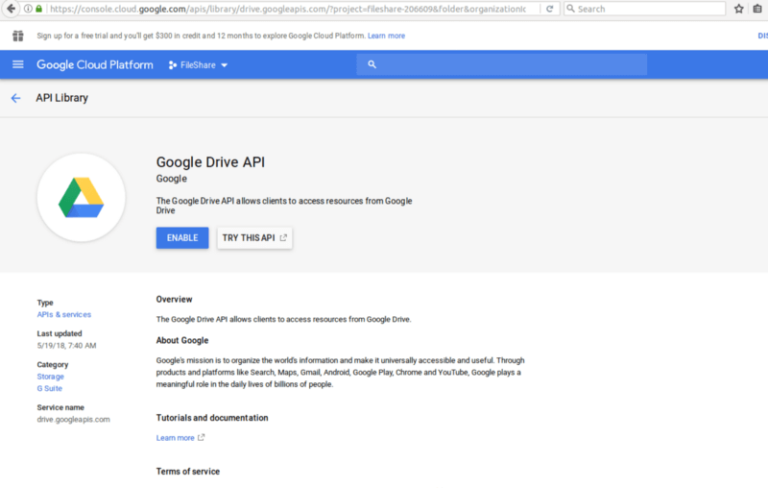This is a low-quality and blurry screenshot of a Google Chrome webpage displaying the Google Cloud Console. At the top of the page, there's a URL address bar containing the address "https://console.cloud.google.com/apis?project?fileshare?206609". To the right of the address bar is a search field with the placeholder text "Search" and a grey magnifying glass icon next to a five-pointed star icon.

Beneath the address bar, there is a white notification banner stating, "Sign up for a free trial and you'll get $300 in credit and 12 months to explore Google Cloud Platform. Learn more." Further down, a purple banner features the text "Google Cloud Platform" in white font alongside a triangle icon and the word "fileshare." Below this banner is another search field with a white magnifying glass icon.

At the top of the main content area is a grey rectangle with the text "API library." The overall interface appears cluttered and difficult to read due to the screenshot's low resolution.